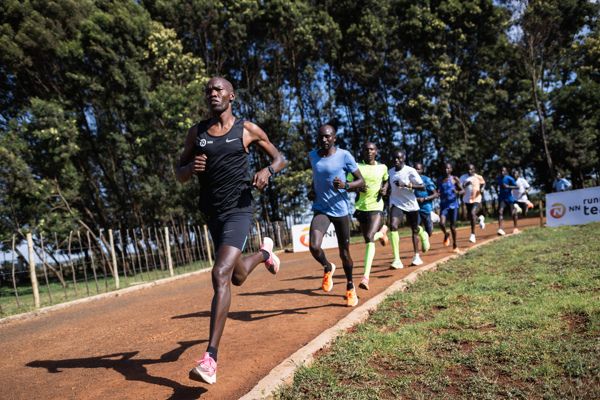The photograph captures a dynamic moment in a track race set against a natural backdrop, likely in Africa. Approximately a dozen African runners are mid-stride on a dirt track with a distinct dark red hue. The track appears to loop in a circular route, evidenced by its curvature and the runners hugging the inner side as they move from right to left, emphasizing the competition. The leading runner, prominently featured in the foreground, wears a black tank top, black shorts, pink sneakers, and black socks, spearheading a diagonal line of athletes. The runners’ outfits are colorful, featuring blacks, blues, greens, oranges, and whites, creating a vibrant scene. The race takes place outdoors, enclosed by a spindly wooden fence that curves along with the track. Beyond the fence, there is lush green grass and a dense line of trees. The daytime sky peeks through the canopy, hinting at good weather. A partial sign with an orange circular logo and some text, partially visible, adds a dash of reference to the scene's specificity. With all participants appearing focused and hardworking, the image beautifully portrays the spirit of athleticism and competition in an open, rustic setting.